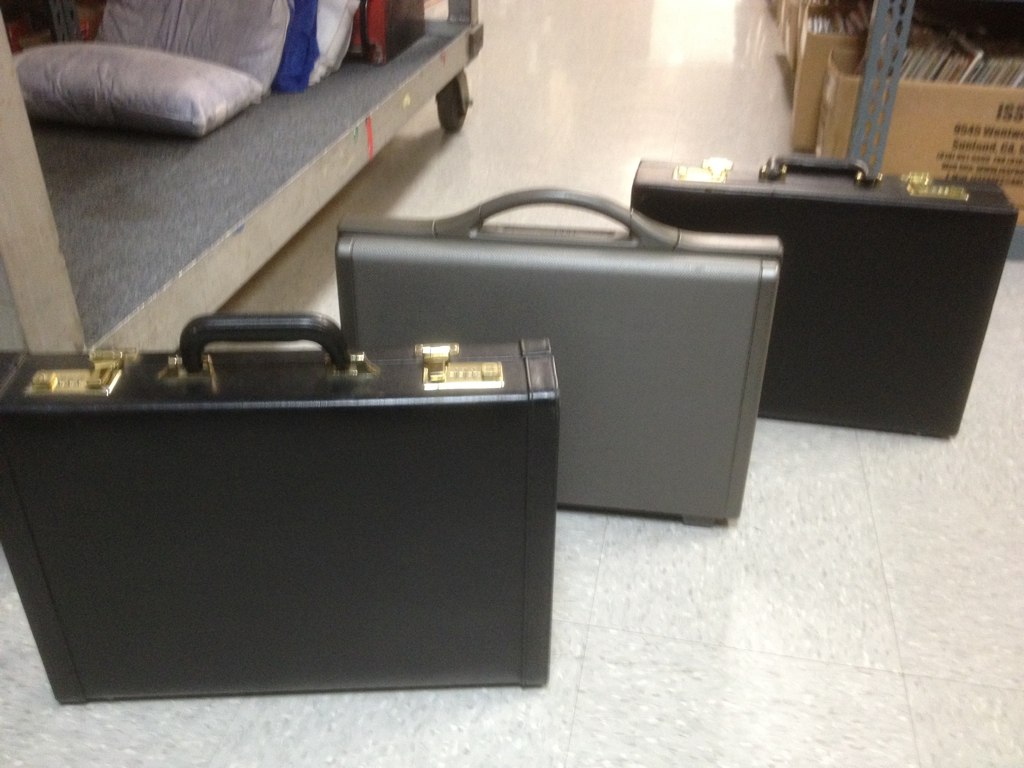In the photograph, we observe a warehouse or thrift shop-type setting. Central to the image are three briefcases arranged diagonally to each other on the floor, clearly reflecting light. The first and third briefcases are nearly identical, featuring black leather material, gold brass locks, combination keypads, and black handles — although one handle is upright while the other is folded. The second briefcase, situated between the black ones, is grayish-silver with a silver trim and a single gray handle, noticeably smaller and thinner than its neighboring cases. In the upper left corner, a metal shelving unit holds packages wrapped in plastic bags and a variety of colored pillows—red, white, blue, and gray. The right side of the photo reveals another metal shelf that seems to serve as a storage area with a couple of cardboard boxes filled with what appear to be vinyl records. The setting and items suggest an environment used for storage or possibly a thrift shop.